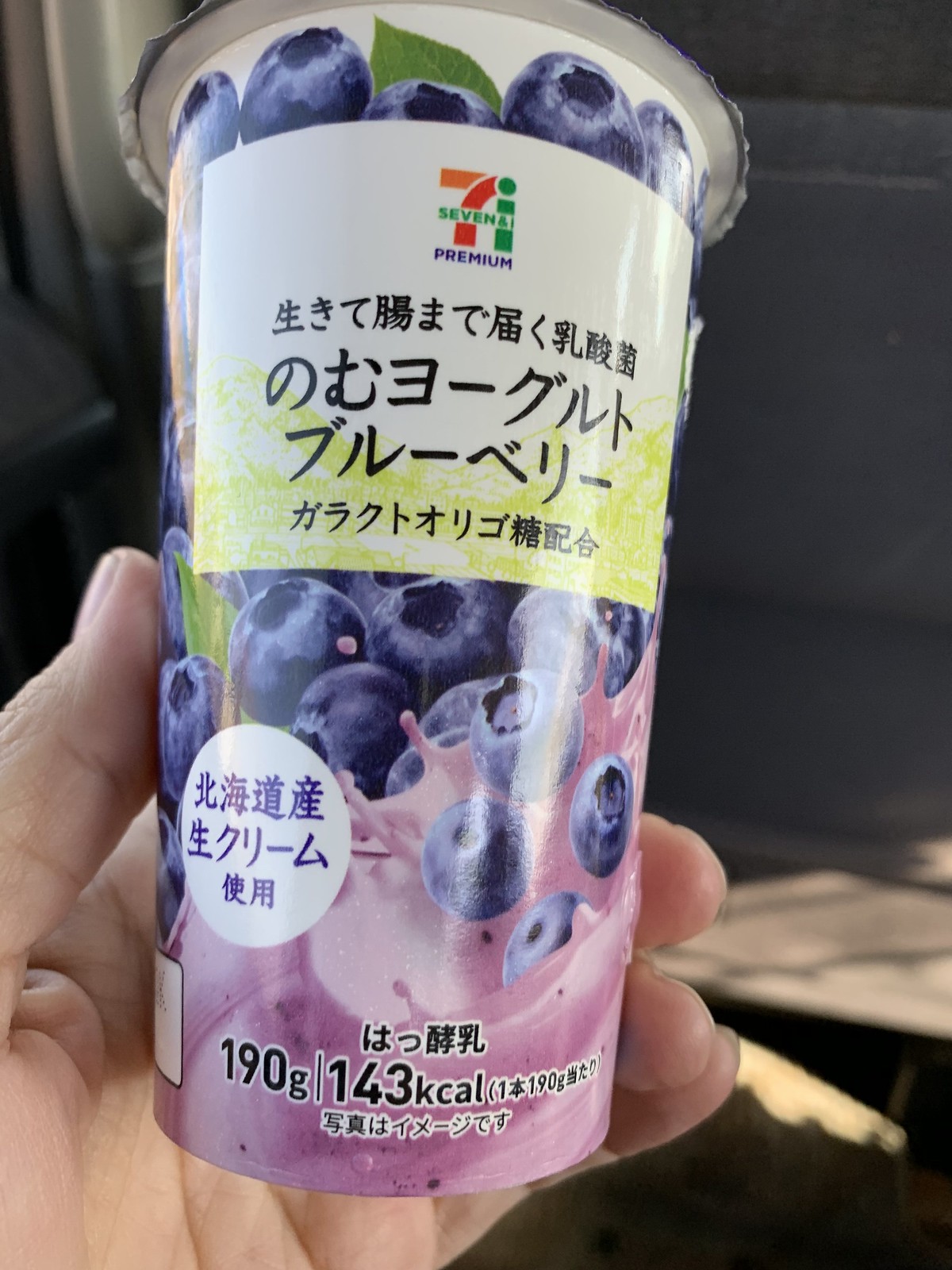The photograph features a close-up view of a white plastic drink container prominently displayed, held in the left hand of the individual. The palm, thumb, and a couple of fingertips of the hand are visible in the bottom left-hand corner. The background, an indistinct blend of gray and brown tones, suggests the photo may have been taken inside a vehicle or plane. The 7-Eleven item is the focal point, adorned with a detailed label showcasing a visually appealing backdrop of blueberries, with some seemingly splashing into a purplish, light lavender liquid at the bottom. The top of the label features the recognizable "7 and I Premium" logo, accompanied by Asian characters, likely Japanese or Chinese, providing additional product details. A circle with more Asian text is situated on the label, and at the very bottom, in black font, the label states "190 grams" and "143 K calories."